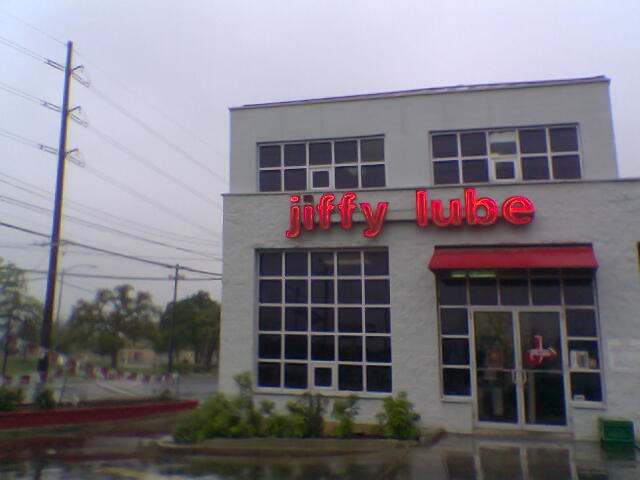The image depicts an outside view of a Jiffy Lube business situated in a gray, two-story building with a smaller second story. The establishment features a red neon sign at the top, which notably has a missing dot on the "i." A red awning is present above the closed double doors. The windows, which are tinted and composed of many small panes, add to the building's aesthetic. The scene suggests recent rainfall, as the sidewalk and road are shiny and reflective, and the overcast sky enhances the gloomy atmosphere. A trash can, gray-brown and square-shaped, is positioned at the bottom right of the image. There is also a strip of greenery with grass and shrubs in front of the window to the left. In the background, to the left, you can see additional parking lots, buildings, and several large trees, with a notably large power line interspersed among them.